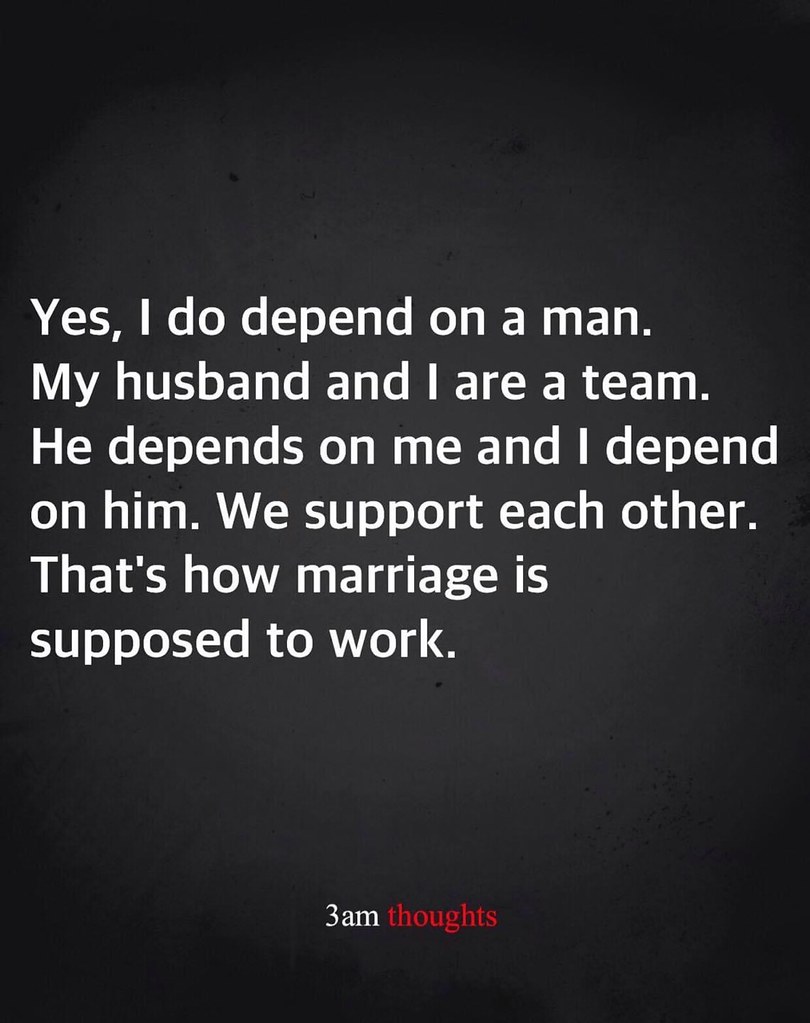The image is a minimalist, black-and-white graphic design with a touch of red for emphasis. The background is a solid black rectangle, and at the center is a left-aligned, six-line block of white text. The text reads: "Yes, I do depend on a man. My husband and I are a team. He depends on me, and I depend on him. We support each other. That's how marriage is supposed to work." Below this, at the bottom center, is the logo "3AM Thoughts," with '3AM' in white and 'Thoughts' in red. The overall style is reminiscent of an inspirational social media post or motivational poster, designed to convey a message about mutual support in marriage.